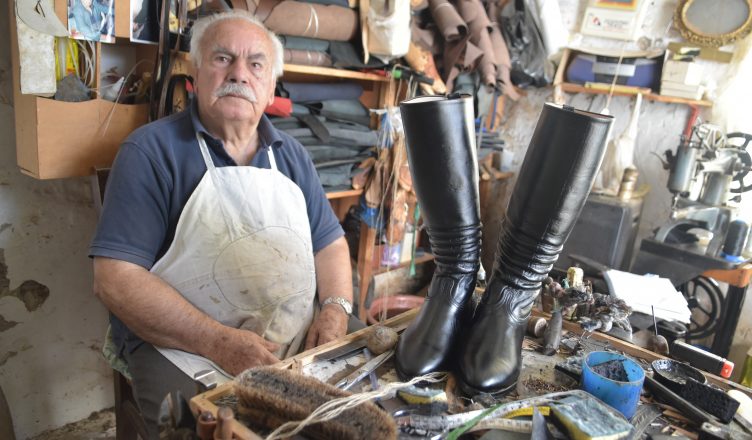In a cluttered cobbler shop, an elderly Caucasian man with receding white hair and a thick white mustache sits on the left side of the frame, wearing a blue short-sleeved polo shirt and a white apron covered in brown stains and smudges. He has a silver watch on his left wrist and stares directly into the camera with a serious expression. In front of him, on a wooden table, lies a pair of shiny black women's boots alongside various tools and materials: a white measuring tape, a blue cylinder possibly containing ink, a tan brush deeply stained with black ink, and other scattered supplies. The background reveals a chaotic scene with several wooden shelves piled with bags and materials, a white wall with damage on the left, a sewing machine placed on a metal surface to the right, and a golden mirror hanging on the wall above the sewing machine. The overall impression is of a workspace overflowing with the tools and remnants of the cobbler's trade.